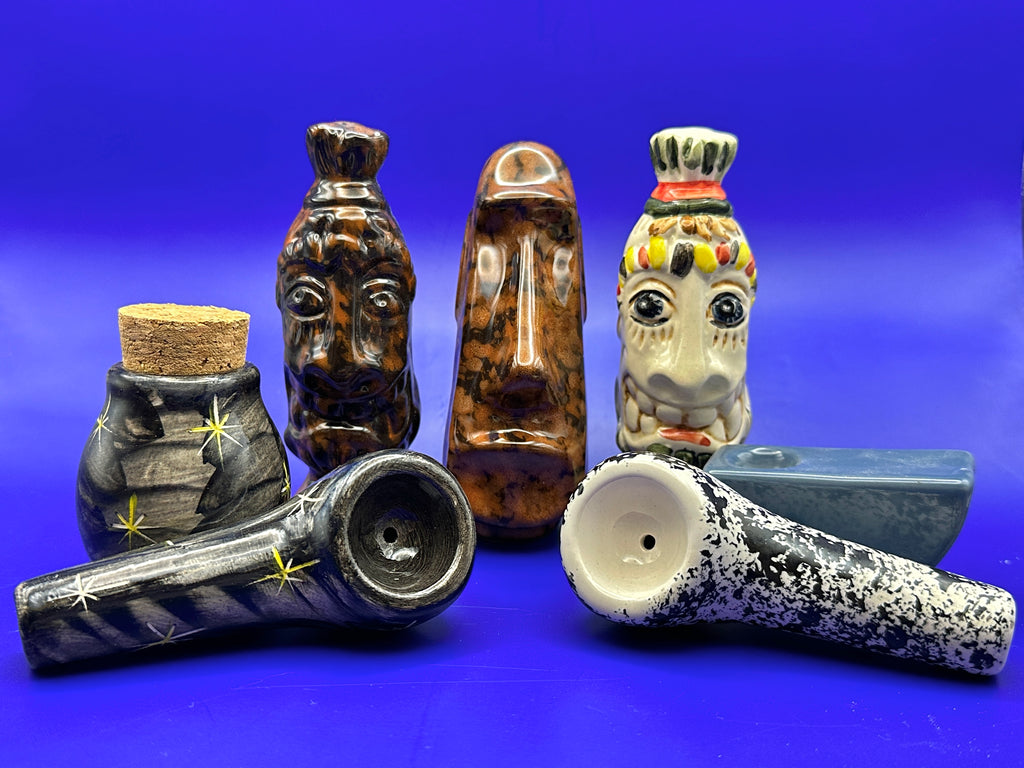The image depicts seven distinct objects set against a blue and purple background, each appearing to be intricately detailed and evocative of tribal craftsmanship. Predominantly made of ceramic, these objects include two smooth, shiny pipes possibly used for smoking, and a small, dark gray container adorned with yellow star designs and sealed with a cork, likely intended for holding herbs. Additionally, there are several colorful decorative figures, each uniquely crafted. One figure is reddish-orange and brown, while another is orange and black. A third figure is white with orange, yellow, and brown accents, showcasing visible teeth, and a bluish item stands in front of it. There is also a white and blue item, alongside a gray, black, and white patterned object with a cork behind it. The overall arrangement and detailing of these objects give an impression of unique, well-crafted totemic sculptures.